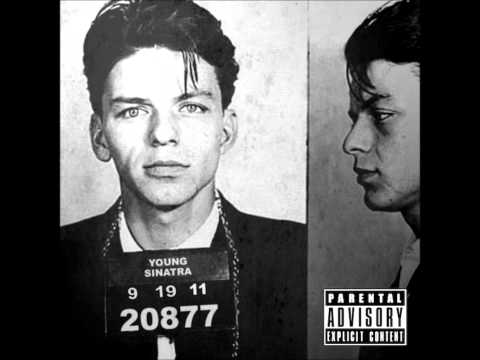The image is a black and white album cover featuring a mug shot of a young man, presumably Frank Sinatra, captured in both a front-facing and profile view. The left side of the image shows his frontal pose with dark hair neatly combed back, except for a single strand hanging over his left eye. He has a clean-shaven, handsome Caucasian face, and wears a black suit jacket over a white collared shirt. Around his neck, there is a black sign with white text reading "Young Sinatra," followed by the date "9-19-11" and the number "20877". The right side of the image features his profile, emphasizing the same neatly combed hair and formal attire. Beneath this side, a rectangular "Parental Advisory: Explicit Content" label appears prominently, with alternating black and white bars and text. The overall composition of the image, side-by-side photographs, and the advisory label suggest it is designed to mimic a police photograph, contributing to the album's thematic aesthetic.